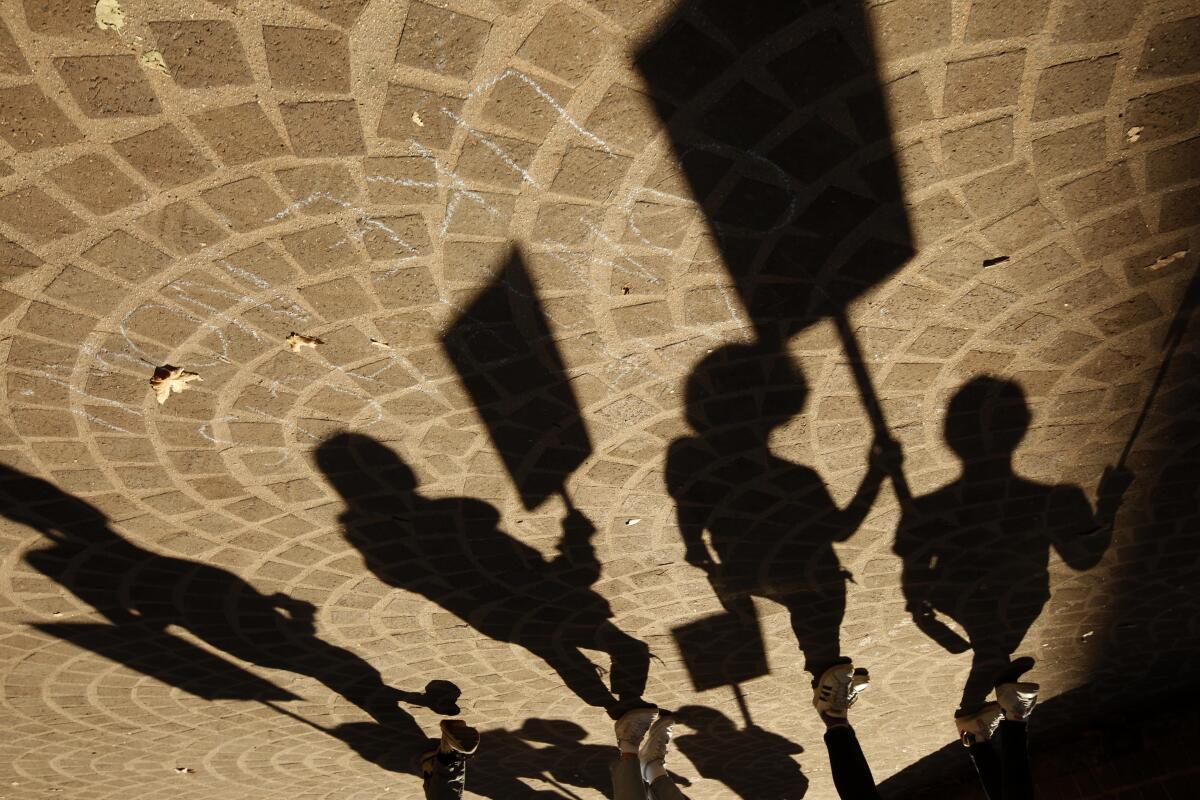The image appears to be a realistic photograph taken upside down, showing a unique and somewhat disorienting perspective of a protest march. The ground, resembling a cement tiled plaza with darker brown tiles and scattered yellow leaves, serves as the backdrop. The ground also features some faint blue chalk writing, including the word "like." Prominently, there are shadows and silhouettes of six people, although four are most clearly defined, projected onto the ground. These people appear to be holding large rectangular protest signs, mounted on sticks or staffs, creating a powerful visual of a demonstration. The visibility of their feet, most wearing white shoes, and the presence of features like an afro and a female figure, add to the realistic detail of the scene. Light from behind the protesters creates elongated shadows, emphasizing the protest signs they hold aloft in this evocative image.